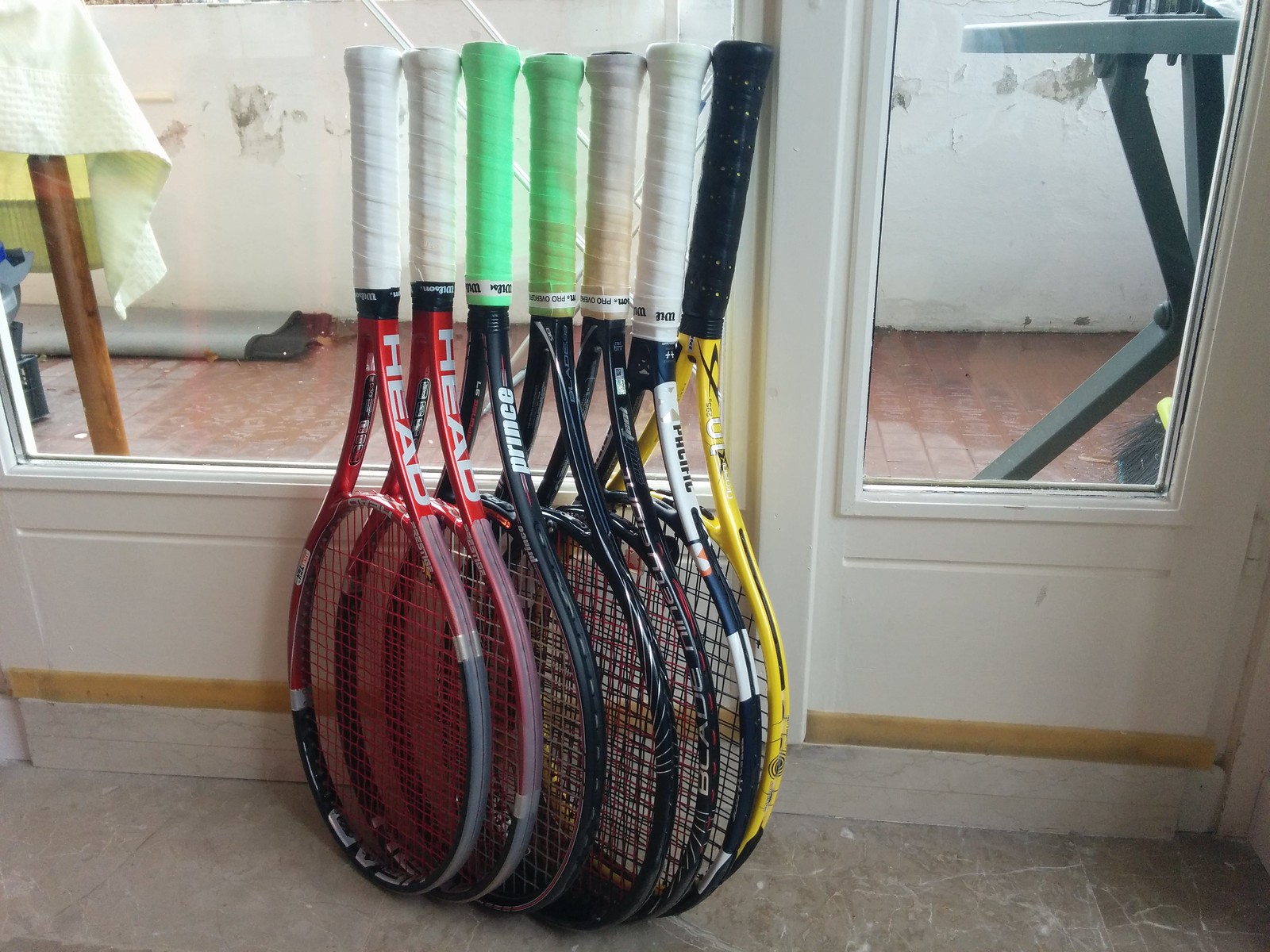In this detailed photograph taken indoors, likely within a home, the scene captures a collection of seven tennis rackets standing upright against a glass wall or window with white trim. The room in the background reveals reddish-brown tile flooring and white walls that appear dingy with some visible gray marks. The rackets are positioned closely together, with their heads only an inch or two apart. The handles display a variety of colors: two rackets have white handles, two have neon green handles, one has an off-white handle, and another has a black handle. The brands of the rackets are diverse, including recognizable names like Head, Prince, and Pacific, although some brands are not clearly identifiable.